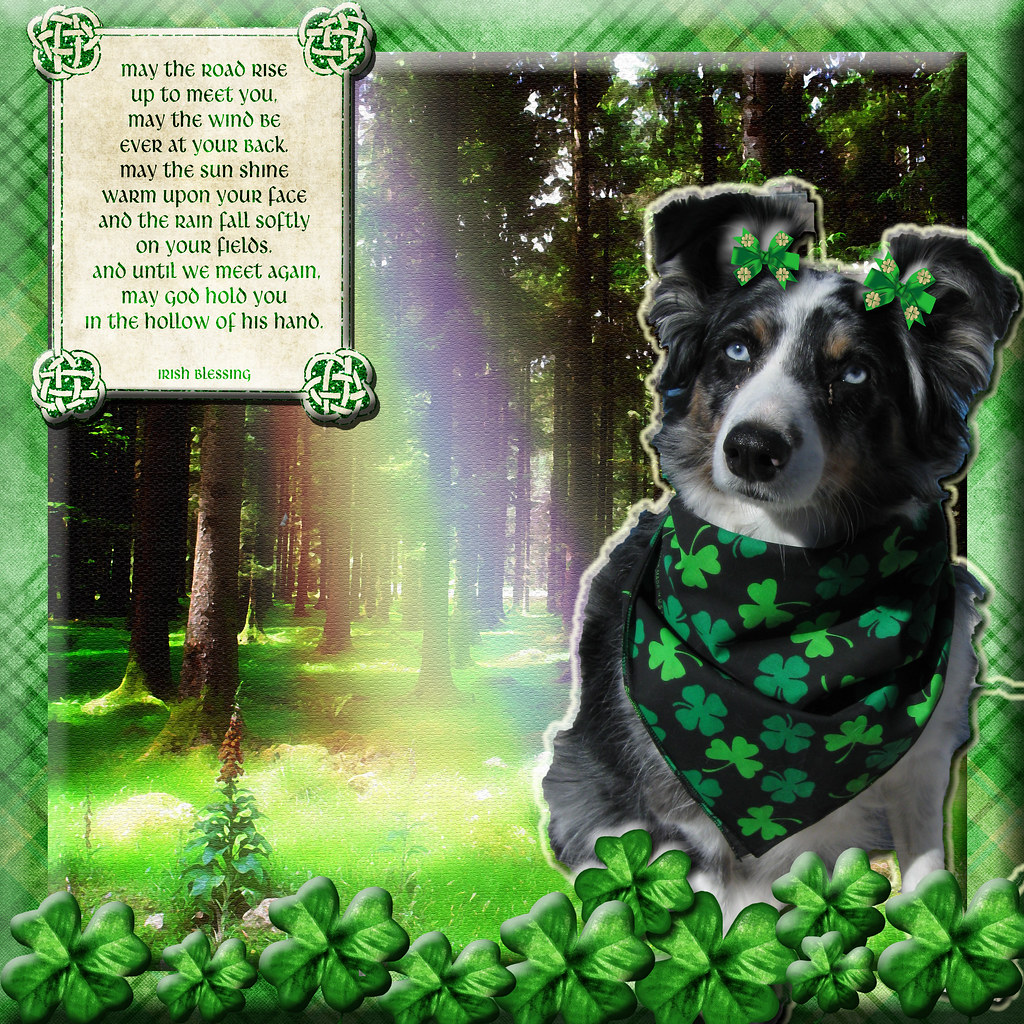This vibrant St. Patrick's Day-themed image features a striking dog prominently positioned on the right side. The backdrop is a lush forest bathed in sunlight with a glimpse of a rainbow adding a touch of magic to the scene. The dog, possibly a Husky or Collie, boasts captivating blue eyes, a black nose, and a uniquely patterned fur that includes a white snout, a splash of white on its forehead, and subtle brown specks. Adorning the dog's ears are charming green bows, while a black scarf patterned with green clovers is wrapped around its neck, enhancing the festive spirit.

The image is bordered by a green frame with darker green lines intersecting in a crisscross pattern, resembling a picture frame. At the bottom, more green clovers are artistically arranged, reinforcing the St. Patrick's Day motif. In the upper left-hand corner, a piece of paper with Celtic symbols in each corner displays a traditional Irish blessing in green text: "May the road rise up to meet you, may the wind be ever at your back, may the sun shine warm upon your face and the rain fall softly on your fields, and until we meet again, may God hold you in the hollow of his hand." This detailed and vibrant composition beautifully captures the essence of Irish celebration and goodwill.